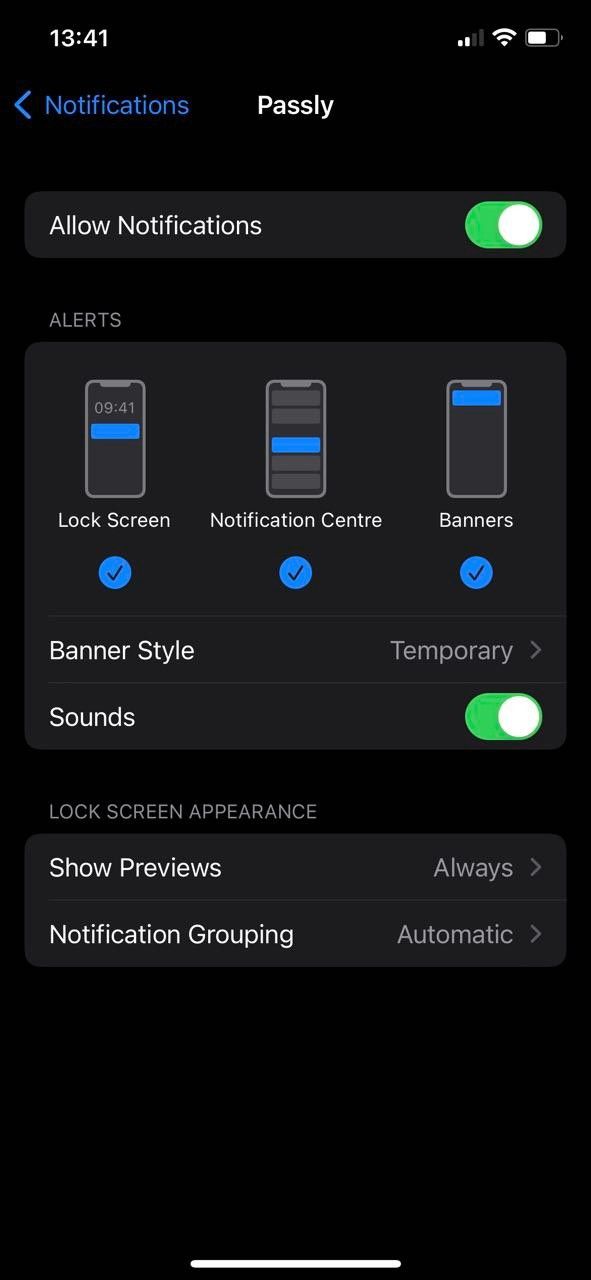The image appears to be a screenshot taken from a mobile phone, captured in night mode due to its black background. In the upper left corner, the time is displayed in white letters as "13:41." The upper right corner features icons for battery status, network signal, and battery level. Just below these indicators, there is a left-facing arrow icon and the word "Notifications" in blue text.

In the center of the screen, the word "Passly" is prominently displayed. Directly beneath this, there is the text "Allow Notifications" accompanied by a toggle switch that is turned on, displaying green color with a white circle.

Further down, the section labeled "Alerts" includes three items:
1. An icon of a phone next to the text "Lock Screen."
2. "Notification Center."
3. "Banners."

Each of these items has a corresponding blue check mark indicating they are selected.

Next, there is a row labeled "Banner Style" written in white text, followed by the word "Temporary" and a right-facing arrow icon. Below this, the text "Sounds" appears accompanied by a green toggle switch with a white circle. The phrase "Lock Screen Appearance" is displayed in light gray beneath it.

Continuing down, there is the label "Show Previews" in white with the option "Always" in light gray, alongside a right-facing arrow icon. Lastly, the section "Notification Grouping" is labeled in white, showing the option "Automatic" with a right-facing arrow icon. The image concludes with a horizontal white line at the bottom.